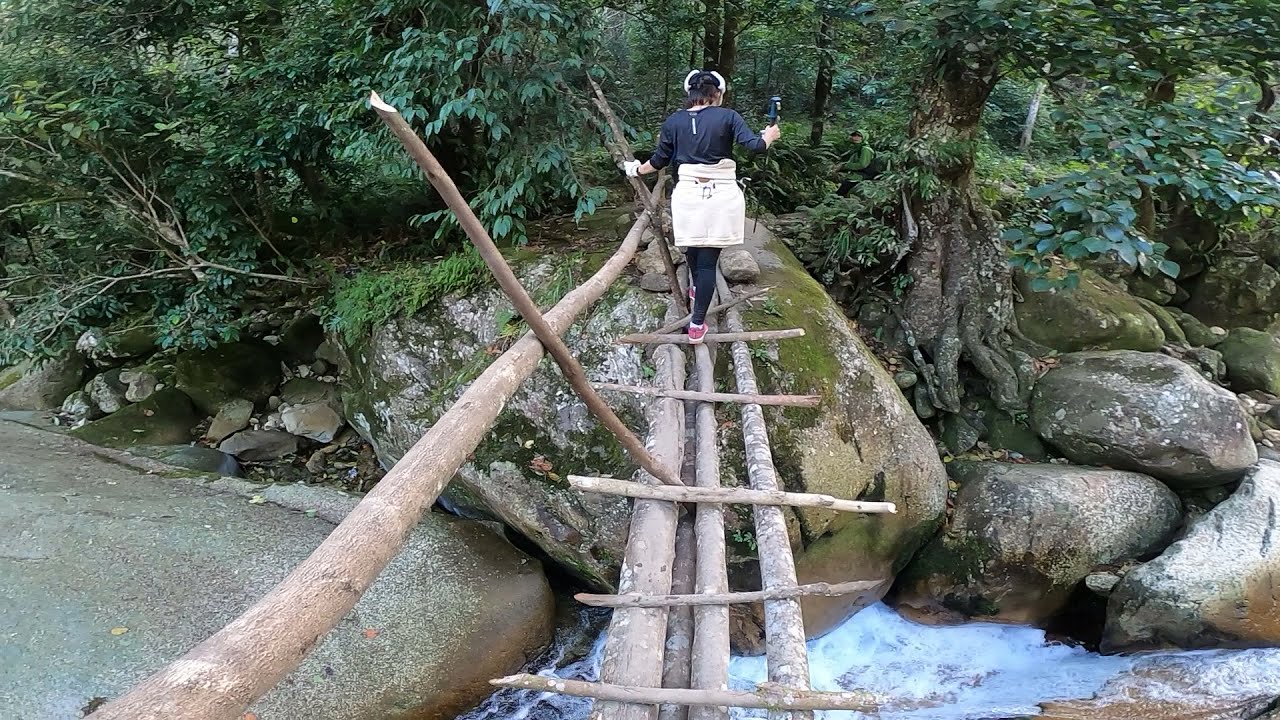In this landscape style photograph taken outside during the day, we see a woman cautiously crossing a crude log bridge over a rocky, rushing river in a lush, wooded area that could resemble the Appalachian Woods in North America. The bridge is constructed from three felled tree trunks laid lengthwise and reinforced with smaller branches placed perpendicularly. The woman, dressed in a dark blue, long-sleeved shirt, black leggings, and red shoes, has a white sweatshirt tied around her waist. She steadies herself with a walking stick in her right hand and grasps the wooden railing on her left. The river below appears swift, framed by large boulders and rock formations, with the trees along the riverbank displaying dense, dark green foliage. The scene is likely set in spring or fall, given the lush leaves and the woman's attire, and the overall lighting suggests a slightly overcast day with no direct sunlight.